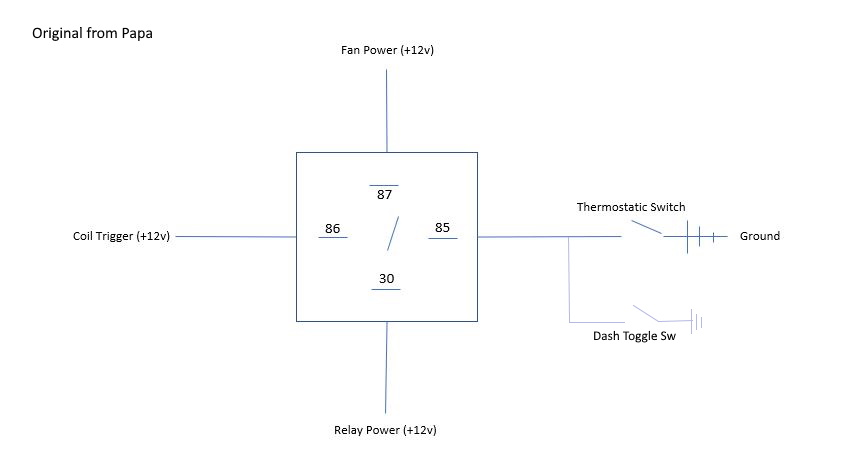The image depicts a detailed schematic chart printed on a white background using blue ink. At the center, there is a square enclosing various two-digit numbers: 87, 85, 30, and 86, arranged in a circular pattern with diagonal blue lines connecting them. Each number has a blue line either above or below it.

From each side of the central square, a line extends outward. The top line is labeled "Fan Power (+12V)." The right line extends towards labels for "Thermostatic Switch," "Ground," and "Dash Toggle Switch." The bottom line is designated "Relay Power (+12V)," and the left line is labeled "Coil Trigger (+12V)."

In the upper left corner of the chart, the text "Original from Papa" is printed, suggesting the source or creator of the design.